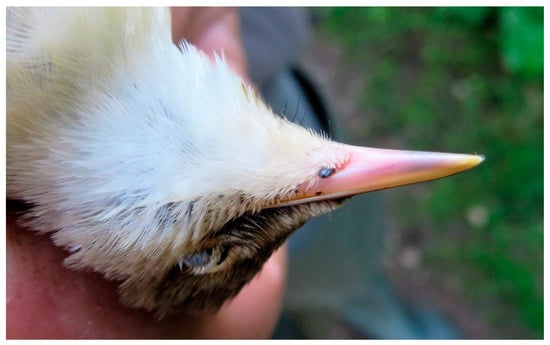This photograph captures a close-up side view of a small bird nestled in a white hand, held upside down, suggesting the bird may be deceased. The bird's head displays a mix of brown and light brown feathers, contrasting with the white feathers on its neck and the underside of its beak. Only one eye is visible, appearing cloudy, reinforcing the impression that the bird is lifeless. The triangular, thin beak is predominantly light pink with a yellow edge. The blurred background hints at an outdoor setting with shades of green and gray, likely grass and possibly a road or path. The image is vertical, with the bird positioned from the top left corner down to the center, emphasizing its delicate features and the underside of its neck.